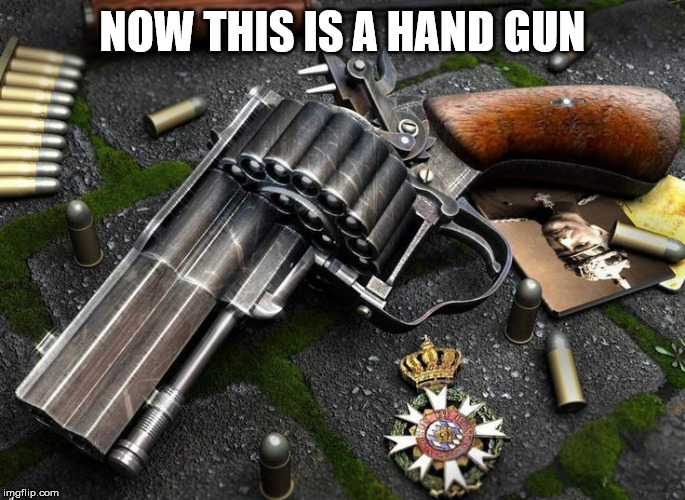The image is a meme with white, all-caps text in the top center, reading: "NOW THIS IS A HANDGUN." The photo is of an unusual, heavily modified revolver displayed on what appears to be a stone-tiled ground with green moss growing between the tiles. The revolver features multiple barrels and a large cylinder capable of holding many bullets, giving it a distinct and exaggerated appearance. Scattered around the weapon are various bullets, some lined up in the top left in a row of approximately ten brass casings with silver-gray tips, and others arranged on the ground. Near the bottom center of the image is a military-style badge adorned with a gold crown, a light green circle with interconnected gold triangles forming V shapes, a red circle with a white background, and intricate gold and blue embellishments. Additionally, there is a rectangle-shaped piece of metal alongside the revolver, possibly a card, which features an upside-down black-and-white portrait of a man in a military uniform, likely from the 1930s. To the right of this piece is a yellow object, further adding to the eclectic collection of items surrounding the revolver.